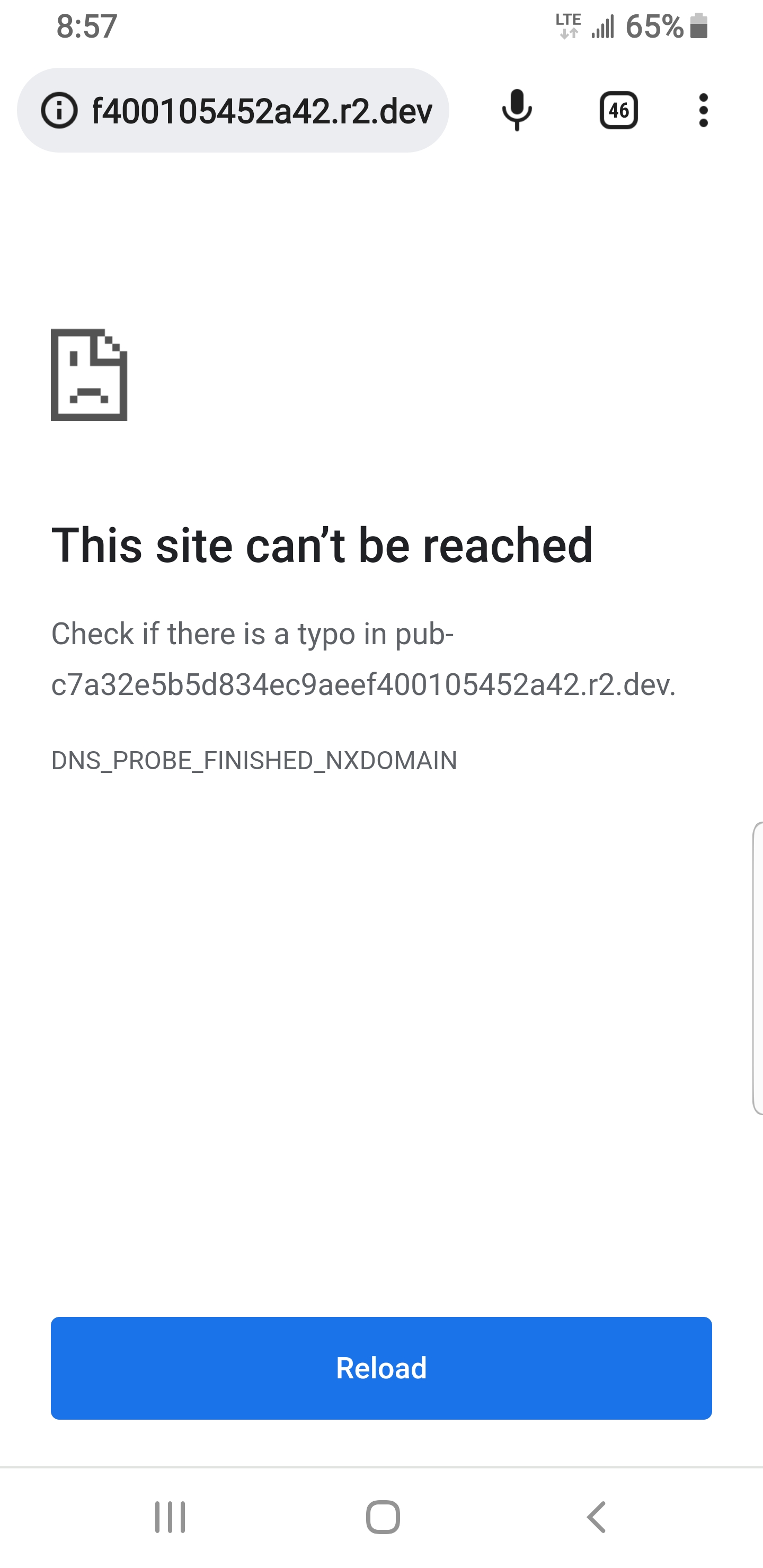This is a detailed digital screenshot taken from a mobile phone at 8:57, with the battery level currently at 65%. On the top right of the screen, a microphone icon is displayed next to a "46" enclosed in a square, followed by three vertical dots. Below this, in bold black font, the message "This site can't be reached" is prominently shown. The text advises checking for a typo in the URL "pub-c7a32e-5b5d-834-ec9aeef-4001054-52a42.r2.dev." The DNS probe has concluded with the result "DNS_PROBE_FINISHED_NXDOMAIN." At the bottom of the screen, a blue and white reload button is evident. Additionally, three gray horizontal lines are visible, possibly indicating a menu or additional options.